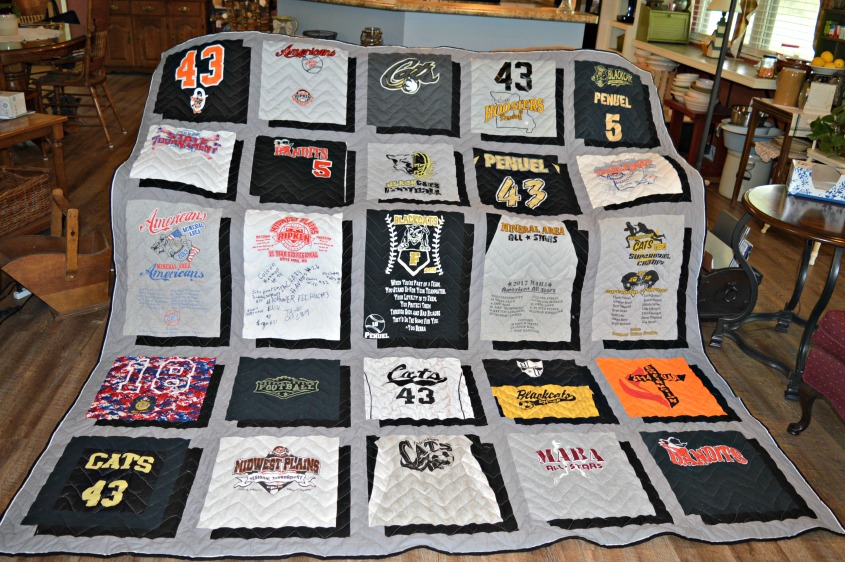This photograph depicts a detailed and carefully crafted sports quilt, likely made from old jerseys and sports t-shirts, prominently featuring the number 43. The quilt, with its patches of various football teams and players, including the "Cats" and the name "Penuel," is set against a gray background and comprises five rows of five equally spaced patches. The quilt is draped over a piece of furniture, with its top half displayed vertically and its bottom half resting on the hardwood floor. In the surrounding environment, the quilt is positioned in a somewhat cluttered living room that blends into a kitchen. To the right of the quilt, a small portion of a red chair and a coffee table can be seen, while further back there is a kitchen area featuring a blue island counter with various objects scattered around and shelves behind the quilt. On the left side of the image, a dining table and a dresser add to the scene, giving the room a lived-in and somewhat disorganized feel.